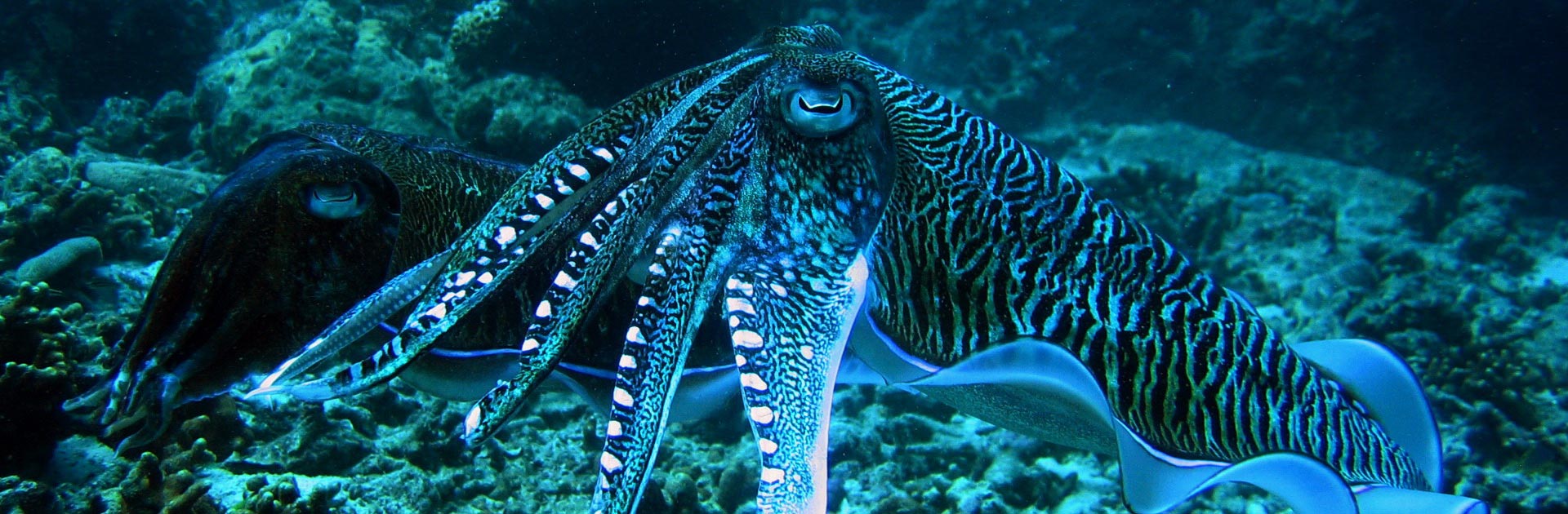This photograph captures a vivid underwater scene at the ocean floor, featuring two cuttlefish amidst a coral reef. The primary cuttlefish, situated prominently in the center, exhibits striking blue and green hues with an intricate pattern of both tiger-like stripes and leopard-like spots in black and dark green, accented by rows of white circles on its tentacles. Accompanied by a slightly darker cuttlefish, possibly black, brown, or green, positioned to its left, the creatures have tentacles extending from their faces and curvy fin-like membranes along their bodies, creating a flowing, almost ribbony appearance. The cool, teal tones of the photograph enhance the serene marine atmosphere, with rocky outcroppings visible in the background, emphasizing the underwater setting.